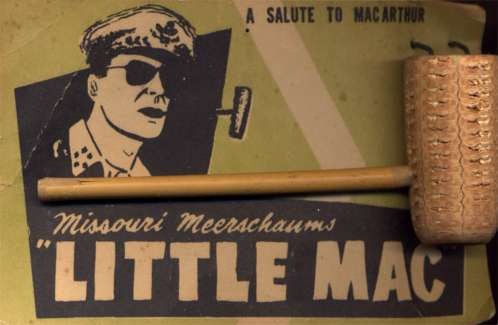The image shows a vintage-style advertisement for a corncob pipe, attached to a thick piece of white cardboard often used for in-store displays. The background is a light avocado or pea green, with a prominent label at the top right corner that reads "A Salute to MacArthur" in dark brown letters. Below this, there is a black-and-white caricature of a man, likely portraying General MacArthur. He is depicted wearing a military hat with an emblem, aviator sunglasses, a white shirt, and possibly a dark jacket, with a corncob pipe in his mouth. To the left of the caricature, the brand name "Missouri Meerschaums" is written in off-white cursive. Underneath, to the right, "Little Mac" is displayed in large block letters. An actual corncob pipe, light beige in color with a long wooden handle and a textured cornwood end, is placed on top of the advertisement, resembling the one shown with the caricature.